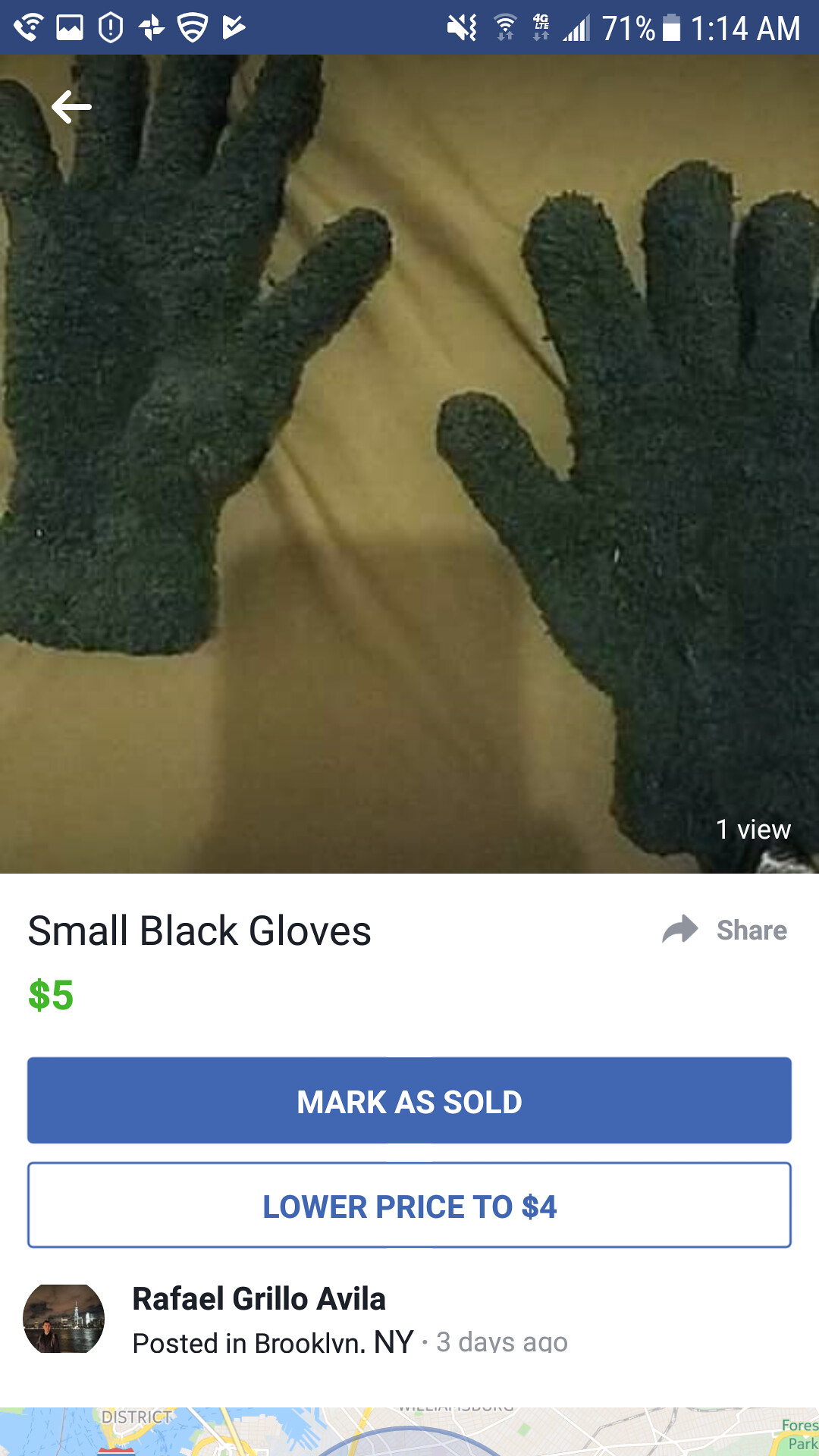This is a screenshot from a Facebook Marketplace post on someone's phone, evidenced by the icons at the top of the image, including the time, battery power at 71%, a four-bar signal indicator, Wi-Fi, and sound settings, along with a phone icon with sound waves on the top left. The primary focus of the screenshot is a low-resolution image of fuzzy black gloves, placed on a beige cloth surface, though somewhat off-center and showing a shadow of the phone used to capture the image. The post is captioned "small black gloves" with a price of $5 in green text. There are two buttons below the description: a blue "mark as sold" button and a white, bordered "lower price to $4" button with blue text. At the bottom of the image, there's a partial map, likely indicating the seller's location, with the seller's details: Rafael Grillo Avila from Brooklyn, New York, posted three days ago.